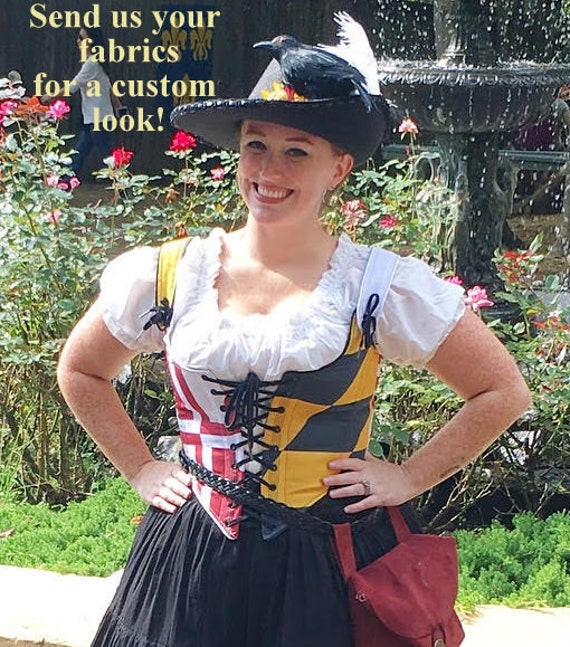This promotional photograph depicts a smiling woman from the waist up, showcasing a customized outfit likely inspired by traditional German attire. The woman, with blonde hair and freckles, wears a vivid ensemble consisting of a black skirt complemented by a braided brown leather belt to which a red satchel is attached on her left hip. Her upper body is adorned with a corset that's creatively split with red and white on the left and black and yellow with diamond patterns on the right, held together by black string. Beneath the corset, she sports a white frilly blouse featuring poofy shoulders and a cutout around the cleavage area. Completing her unique look, she dons a black brimmed hat adorned with a black fake bird, with the left brim elegantly curved upwards. The background reveals green plants, a water fountain, and people strolling, adding a casual, lively atmosphere. Notably, yellow text in the top left corner reads, "Send us your fabrics for a custom look," indicating this photograph promotes custom tailoring services.